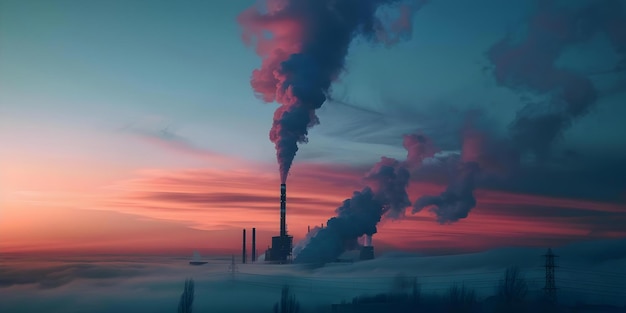The image depicts a large, black industrial building prominently centered against an evocative background. The main structure, likely a factory, is characterized by its three distinct columns, with the central smokestack emitting a heavy plume of white smoke that rises into the sky. The scene captures a significant contrast between the foreground and backdrop. In the foreground, the colors transition from pure white to light blue, suggesting a snow-covered or frosty landscape. The sky behind the building is remarkably vivid, with hues of pink, red, and blue that transition into darker shades, resembling either a sunrise or sunset. The smoke itself appears illuminated by the ambient light, reflecting pink tones. This image, which may be a detailed drawing or poster rather than a photo, meticulously highlights the isolated factory amidst a stark, cold setting, with a streaked, colorful sky that accentuates the industrial activity.